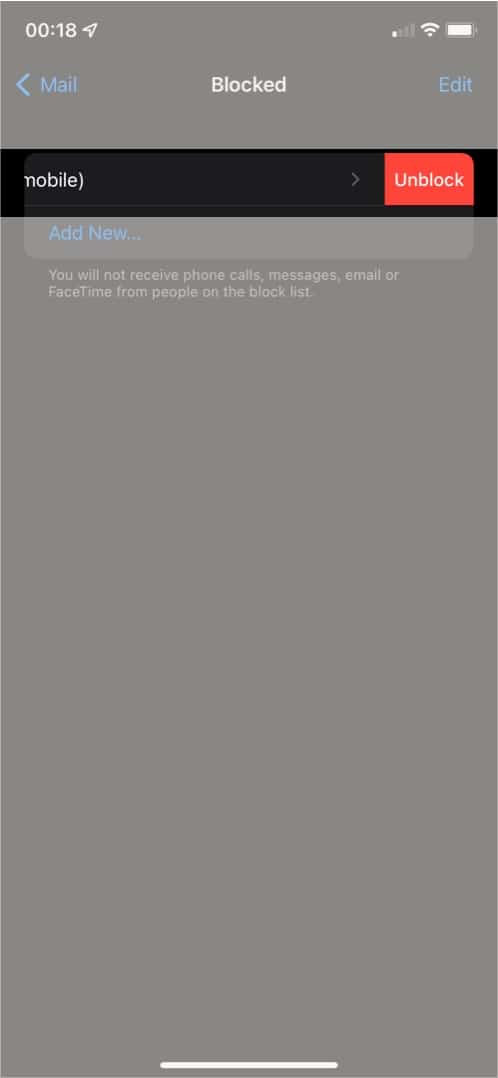The image depicts the screen of a smartphone displaying a website with a light gray background. The phone shows a fully charged battery icon, a strong connection, and the time indicated as 18 seconds. At the top, there's a blue "Mail" icon with a left-pointing arrow. In the center of the page, the word "Blocked" is prominently displayed in large white letters. To the right, there is a blue "Edit" option.

Below this, a horizontal bar spans the width of the screen, featuring the word "Mobile" in white on the left side and a red square with "Unblock" written in white on the right side. Further down, a blue "Add New" option is visible. Additionally, there is a notification stating, "You will not receive phone calls, messages, email or FaceTime from people on the block list," indicating the function of this screen.

The entire phone screen is captured in the image, with nothing shown underneath the aforementioned text. At the bottom, there's a white line, but no further images or text are present. The layout is clean, with clear and concise information focused on the blocking feature.